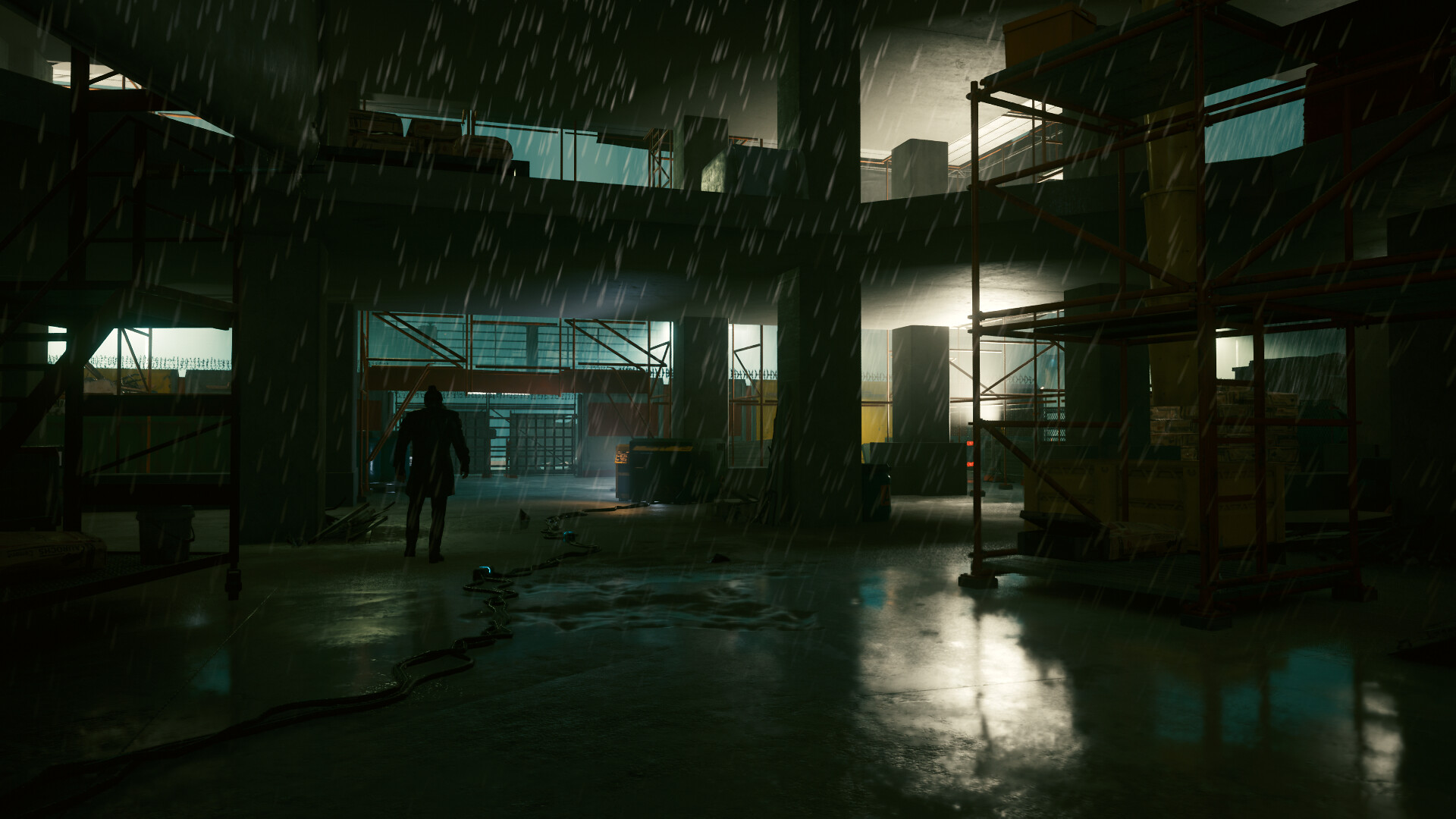In a dimly lit, rainy night scene, the image captures a multi-level cement construction complex, specifically within a parking garage area. The wet ground, reflecting the ambient light, reveals the recently fallen rain. Two stark white lights illuminate both the first and second floors in perfect alignment, casting a stark contrast against the otherwise muted environment. To the right, a blue plastic sheet is conspicuously draped along the back wall, extending up to a window on the upper floor where it’s partially visible. A network of metallic scaffolding stands as a skeletal framework, indicative of ongoing construction, permitting workers to navigate the structure. Distinctly on the left side, the silhouette of a solitary figure is discernible, adding an element of mysterious human presence. Adjacent to this silhouette and slightly leftward, a sturdy beam supports the concrete infrastructure. Above, scattered boxes on the second floor hint at the ongoing nature of the building process, completing the industrial and somber mood of the scene.